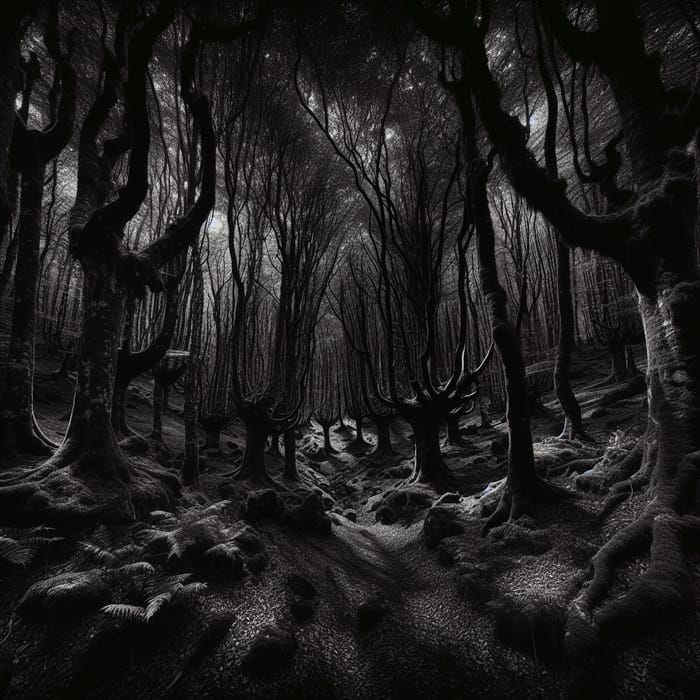This is a black and white artistic drawing of a haunting and desolate forest, possibly created in pencil. The vertically rectangular image lacks any defined border, immersing you in a creepy, nightmarish scene. The forest is filled with irregularly shaped, thin, and lanky trees devoid of leaves, their bare branches stretching skyward. There are no signs of life; even the ground, littered with rocks and what appears to be a dry riverbed, shows no foliage or dead leaves. Towards the left side of the drawing, you can see a bright, round spot that is likely the moon, casting an eerie gray light over the scene. This moonlight breaks through the branches, creating stark shadows on the uneven, dirt-covered ground, adding to the sense of foreboding. The overall ambiance is dark and gloomy, reminiscent of a setting from a horror story where a witch might dwell, amplifying the chilling and lost-in-the-woods theme.